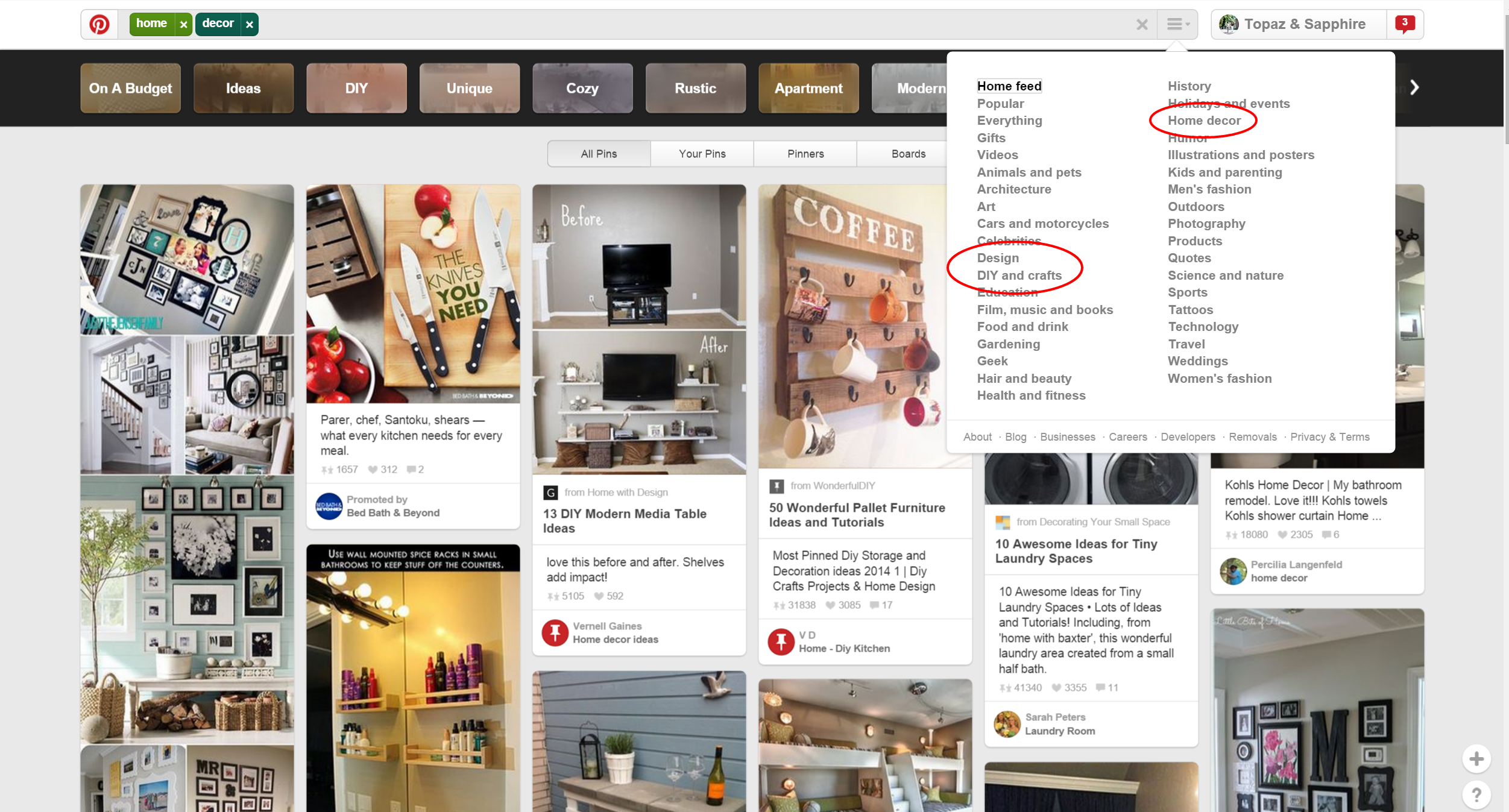This rectangular image, with its long side running horizontally, appears to be a screenshot from Pinterest. It features a white border at the top, which includes the Pinterest logo and a search bar with the terms "home" and "decor." A small pop-up window is open, labeled "home feed," displaying several categories such as popular, everything, gifts, videos, animals, and pets. Within this pop-up, two specific categories - "Design & DIY" and "Home Decor" - are highlighted with red circles.

Beneath the pop-up window is a black horizontal border featuring brownish-gray boxes that list various thematic ideas: On a Budget, Ideas, DIY, Unique, Cozy, Rustic, Apartment, Modern. Below this section, the image showcases a collection of visual suggestions and clickable thumbnails related to home decor and DIY concepts. These visuals portray various interior design elements like shelves, TV stands, artwork, and room arrangements, offering diverse inspirational ideas for home improvement and decoration.